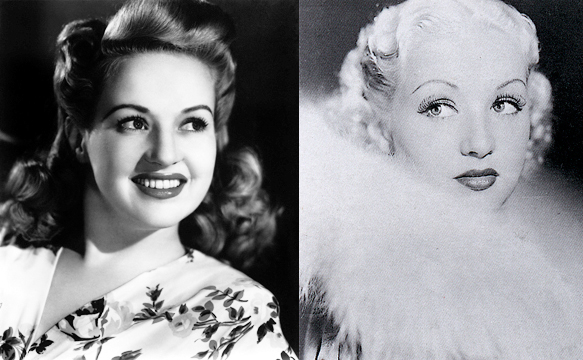The image depicts two black and white photographic portraits of the iconic 1940s film star, Betty Grable. In the left photograph, Betty is seen with dark, curly hair adorned in a floral-print top. She's smiling brightly, her dark lipstick accentuating her teeth, and her eyes gazing slightly to the right. The background behind her is very dark, emphasizing her expressive, joyful demeanor. The right photograph presents a stark contrast. Betty's hair is styled in a close-cropped, white, wavy fashion, and she exudes glamour with a fluffy, white feather boa around her neck, obscuring the lower part of her jaw. Her lips are dark and pursed, and her light-colored, piercing eyes look to the left. The photograph's lighter background complements her sophisticated and almost enigmatic presence. Despite the dramatic differences in hairstyle and expression, both images showcase the timeless allure and versatility of Betty Grable.